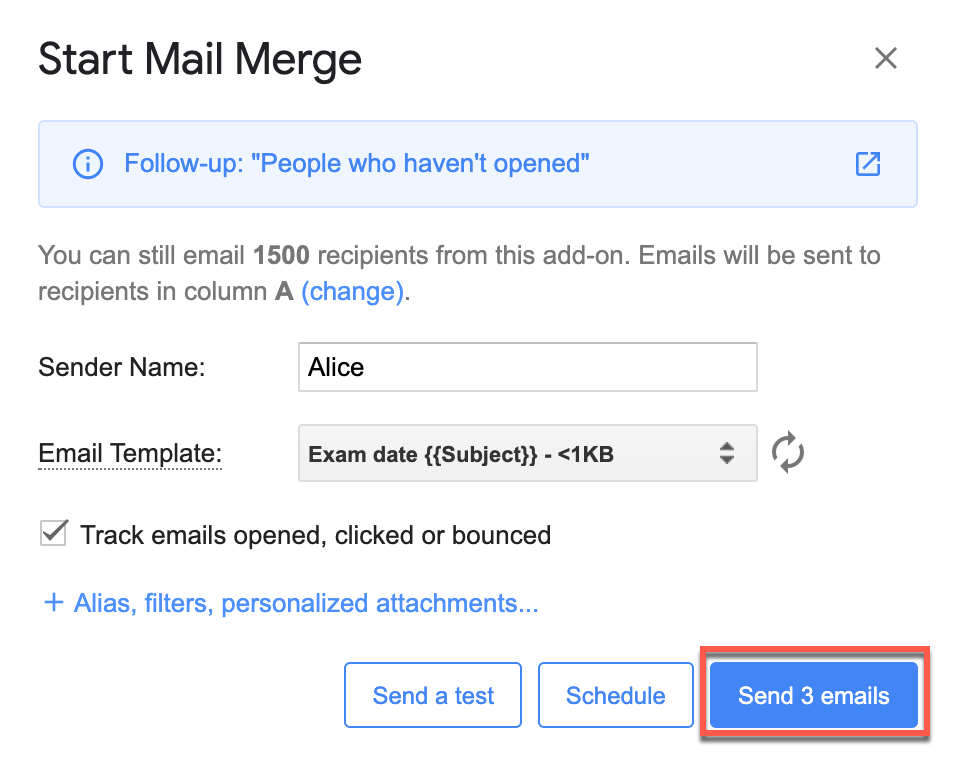This image showcases the interface of an email marketing tool, featuring various functionalities and statistics. The text prominently highlights the option to follow up with people who haven't opened the initial email. It also states that you still have the capability to email up to 1,500 recipients using this specific add-on. The emails are intended to be sent to recipients listed in Column A, with the additional ability to change the sender's name to "Alice". 

Additional features displayed include the use of email templates about exam dates and subjects, with file sizes less than one kilobyte. The tool tracks key metrics such as whether the emails were opened, clicked, or bounced. It also supports the use of aliases, application of filters, and inclusion of personalized attachments. There are options to send a test email, schedule emails, and send up to three emails as part of this process.